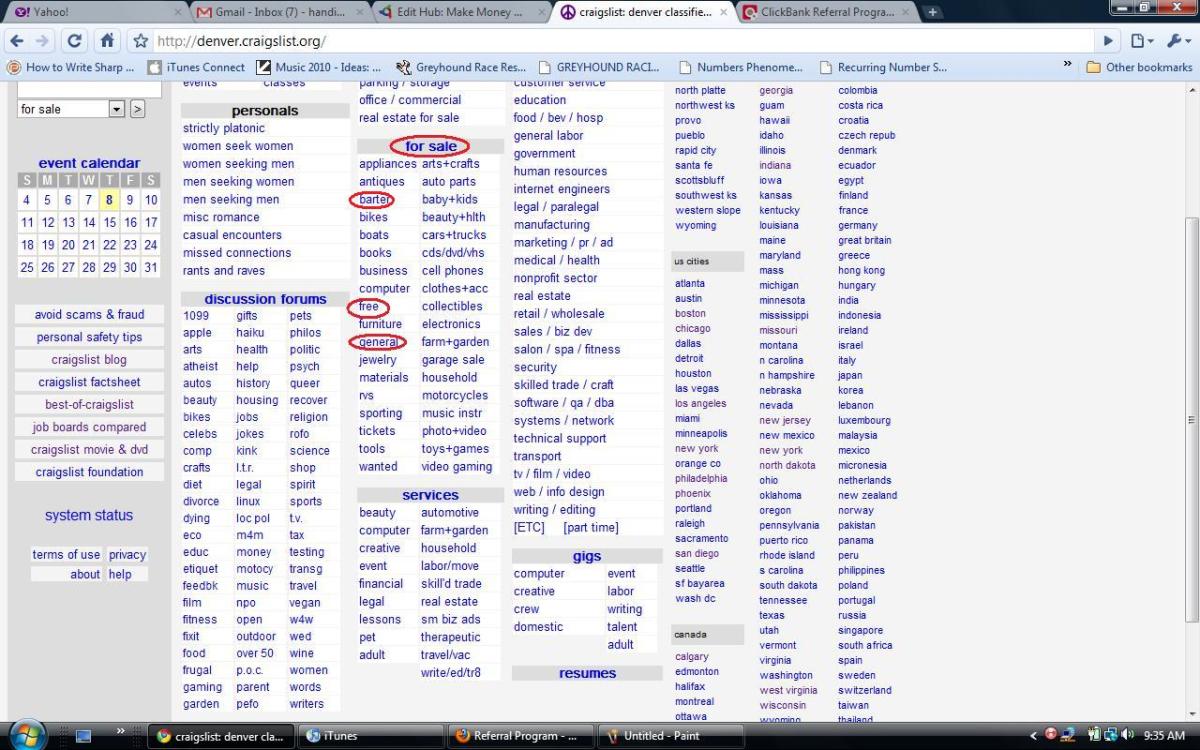This image showcases a webpage with numerous open browser tabs. The tabs at the top are: Yahoo, Google/Gmail, Etihub Make Money, Craigslist Denver Classifieds, ClickBank Referral Programs, and several others unidentifiable as the tabs are blacked out. The browser navigation area includes a left arrow, a right arrow (grayed out), a refresh button, a home button, and a star icon. The URL or address bar is visible but unspecified.

Below the navigation bar, there is a blueprint layout with various text entries: "How to write Sharp," "iTunes Connect," "Music 2010 Ideas," "Greyhound Race," "Greyhound Race," "Numbers Phenomenon," and a partially visible entry ending with "dot dot dot."

A gray sidebar is present on the webpage, featuring several sections and items: a blank space followed by "For Sale," an "Event Calendar" with Thursday highlighted, and "Avoid Scam and Fraud." Additional links in the sidebar include "Craigslist Blog," "Request a Craigslist," "Craigslist Movie and DVD," "Craigslist Foundation," "System Status," and "Terms of Use." Further sections mentioned are "About Privacy and Health," and categories such as "Personals," "Discussion Forums," and "For Sale."